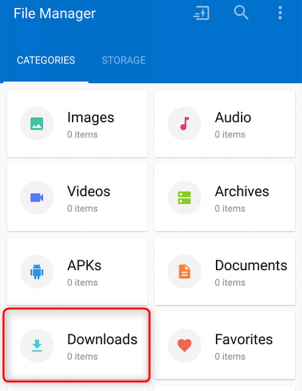The screenshot captures the settings area of a website, specifically showcasing the "File Manager" section, which is prominently displayed at the top left corner on a blue bar. The interface is divided into two main sections: "Categories" and "Storage". The "Categories" section is currently highlighted, indicating that it’s the active view. Within the "Categories" section, various options are listed, including Images, Videos, APKs, Downloads, Audio, Archives, Documents, and Favorites. Notably, the "Downloads" option is distinctly bordered in a red line, drawing special attention to it.